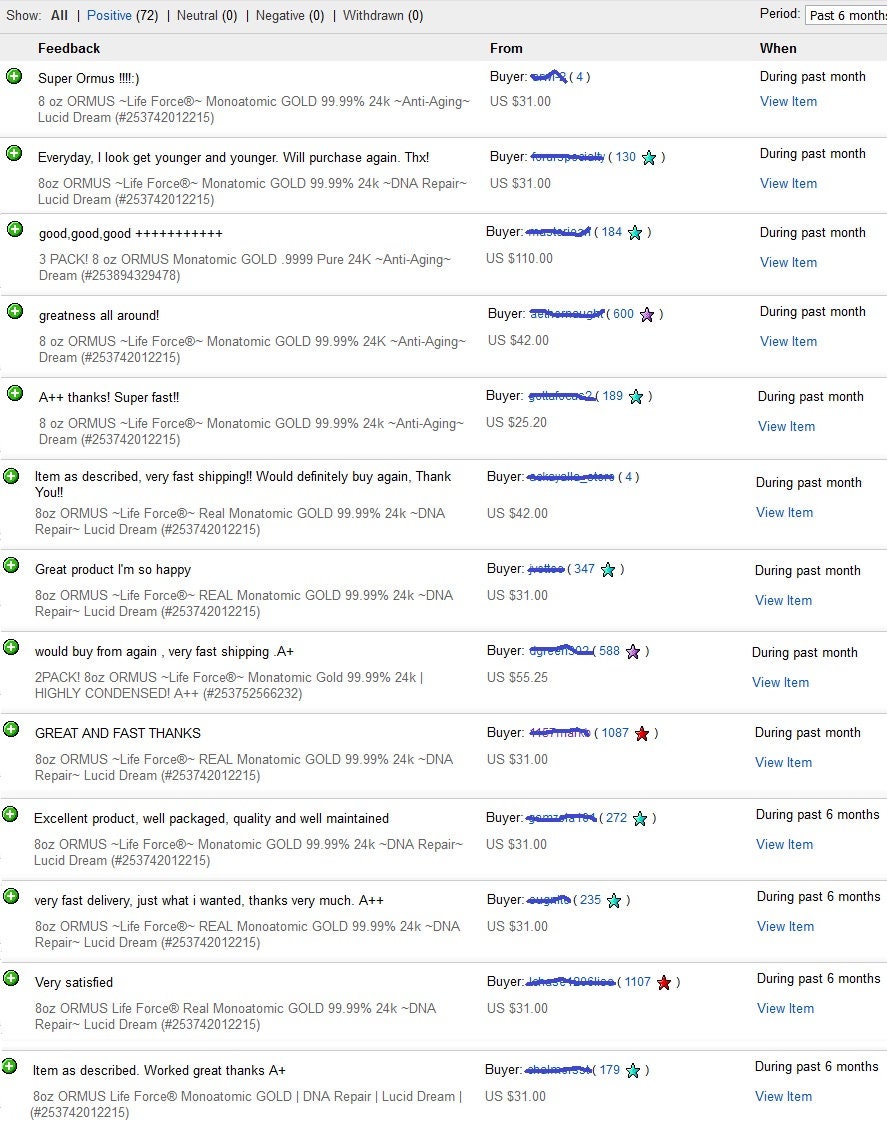**Caption:**

Displayed at the top of the image are summarized customer sentiments over the past six months: 72 positive, 0 neutral, 0 negative, and 0 withdrawn. 

Highlighted is the "8 oz Ormus Life Force Monoatomic Gold 99.99% 24 Karat Anti-Aging Lucid Cream," priced at $31 within the past month, with a prompt to view items. 

Customer reviews emphasize satisfaction with statements like:

- "Every day I look younger and younger. Will purchase again. Thanks!"
- "Good, good, good, and a bunch of pluses."
- "Greatness all around. Pluses thanks."
- "Super fast item as described, very fast shipping. Would definitely buy again. Thank you!"
- "Great product, I'm so happy!"
- "Would buy from again, very fast shipping."
- "Excellent product, well packaged, quality and well maintained."

Each review reflects high praise for the product’s effectiveness and the efficient service provided.